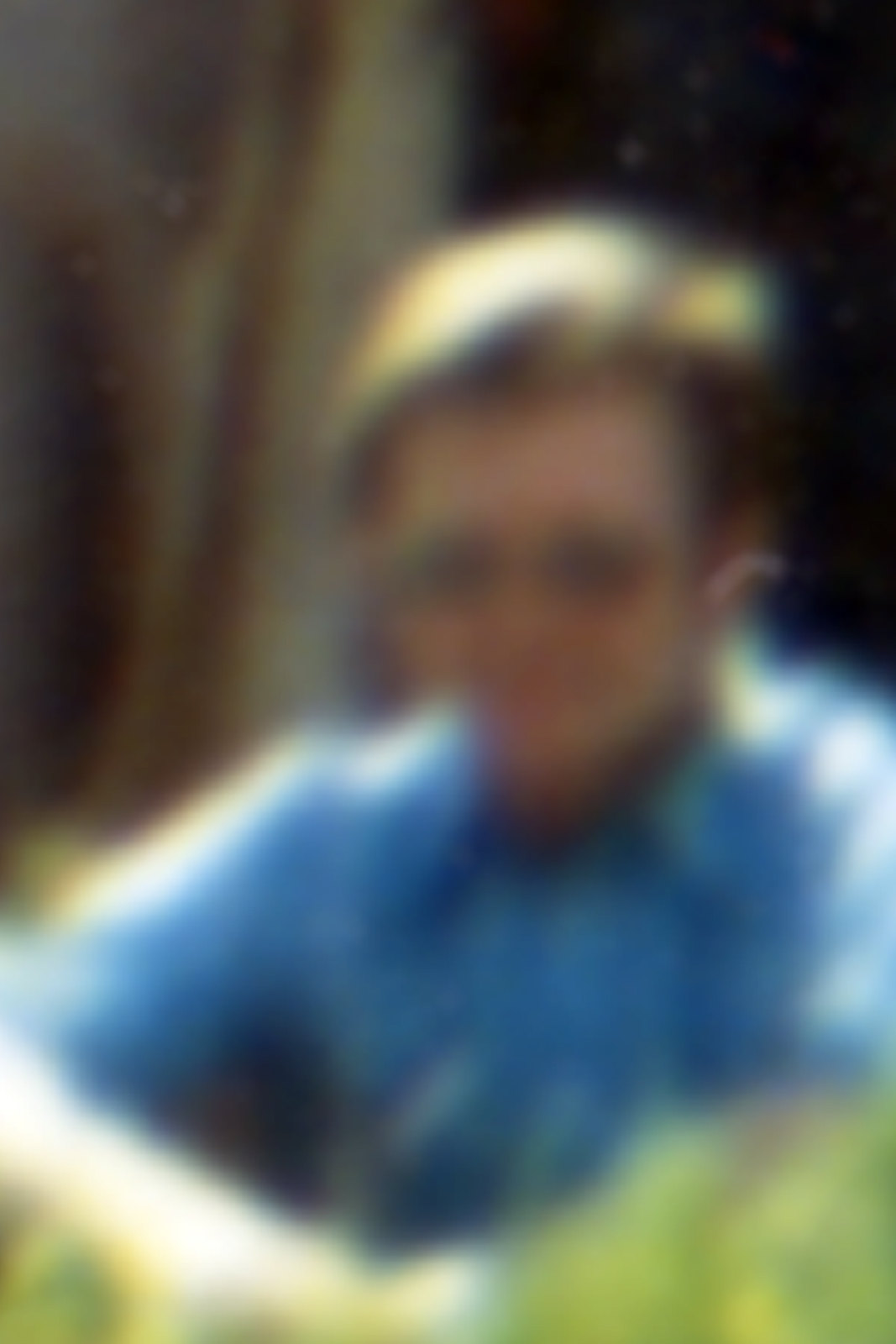In a very blurry and out-of-focus outdoor image, a man is seated with his elbows resting on his knees. He has short brown hair and is wearing a blue, button-down shirt with a collar. The sleeves of his shirt are either short or three-quarter length. The man appears to be wearing tinted glasses, possibly sunglasses, and his upper body is illuminated by sunlight. The background is indistinct but shows some green, likely bushes, along with blurred patches of black and light brown, which might be trees or other natural elements. The overall low quality of the photo makes it difficult to discern finer details of his features or the exact surroundings.